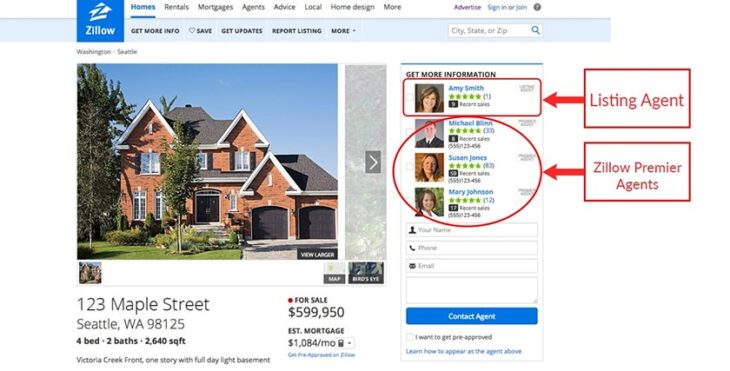A detailed, cleaned-up caption for the image:

"This image is a screenshot of a Zillow webpage featuring a real estate listing in a landscape rectangular format, suitable for viewing on a laptop or desktop monitor. The page is designed with a dual-row header. The top row has a white background and includes the Zillow logo on the left, which consists of a blue circle containing a white house with a blue 'Z' and the word 'Zillow' beneath it in white. 

To the right of the logo, there are navigation options: 'Homes' (highlighted in blue with a thick underline), 'Rentals,' 'Mortgages,' 'Agents,' 'Advice,' 'Local,' 'Home Design,' and 'More' (all in gray). Further right, the options 'Advertise,' 'Sign In' or 'Join,' and a gray information icon (circle with a question mark) are listed.

The bottom row of the header has a light blue background with five sections in all caps: 'GET MORE INFO,' 'SAVE' (with a heart icon), 'GET UPDATES,' 'REPORT LISTING,' and 'MORE' (with an arrow icon). There is a search bar to the right, prompting users to enter a city, state, or zip code, accompanied by a magnifying glass icon.

Below this header, the main content displays the listing details. In light gray text on the upper left, the location is indicated as 'Washington > Seattle.' A large image of a brick, multi-story house with gray slanted roofs, surrounded by grass and trees, is prominently shown. The address below the image reads '123 Maple Street, Seattle, WA 98125.' The property specifics are listed beneath: '4 bed, 2 baths, 2,640 SQFT.' The price is displayed to the right as '$599,950,' marked with a red dot and labeled 'For Sale.' Underneath, it details the estimated monthly mortgage as '$1,084/mo.'

To the right segment of the page, a section labeled 'Get more information' presents headshots of four real estate agents. The agents, all depicted from the shoulders up, are listed in the following order: Amy Smith (top, five green stars, one review), Michael [Last Name Unreadable] (five stars, 32 reviews), Susan James (five stars, 83 reviews), and Mary Johnson (five stars, 12 reviews). The latter three have their phone numbers listed beneath their star ratings.

Amy Smith is identified as the listing agent with a red rectangle and arrow pointing to her image. The other three agents are collectively marked as 'Zillow Premier Agents' within a red circle. Below this section is a contact form with fields for entering name, phone, email, an optional comment field, and a blue 'CONTACT AGENT' button."

This cleaned-up caption provides a thorough and organized description of the Zillow webpage, making it easy to visualize and understand the elements and layout described.